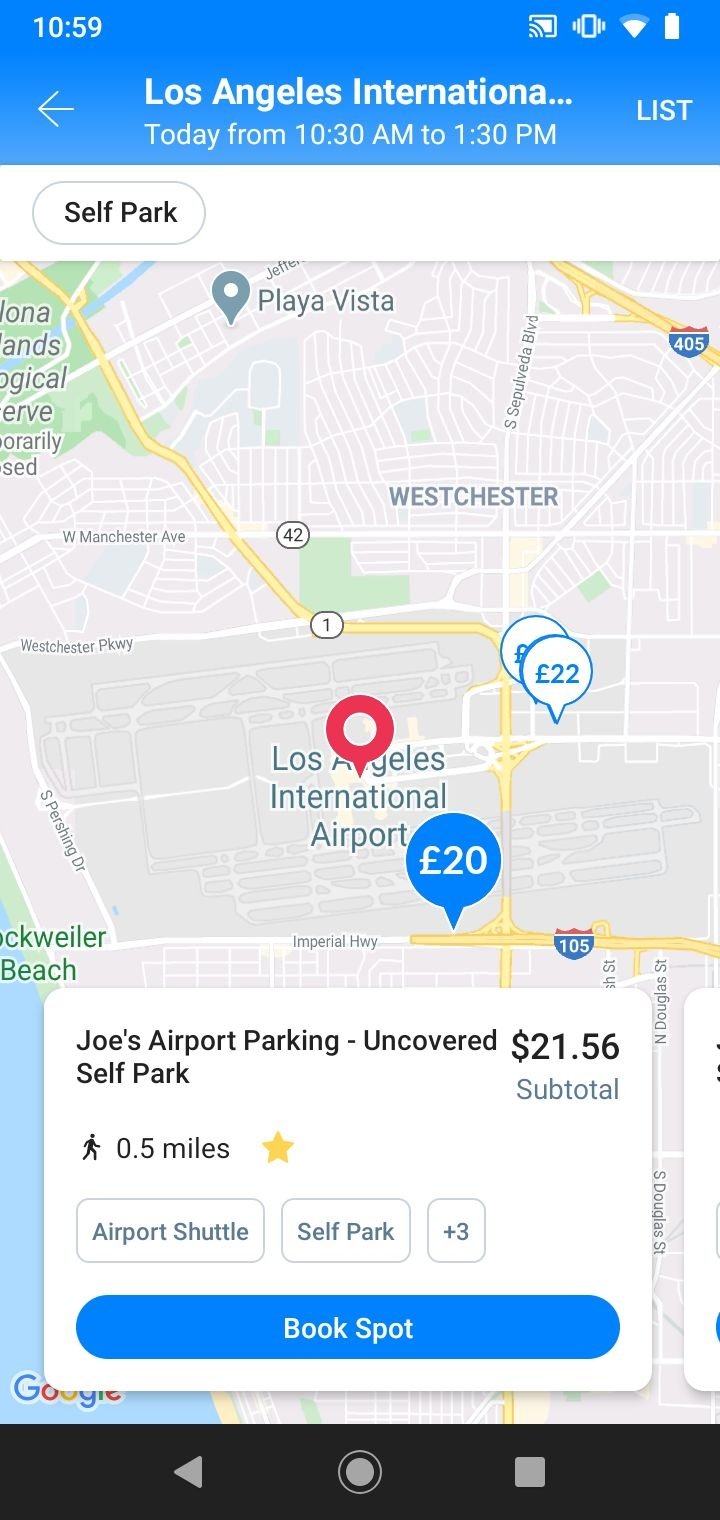The image displays a detailed screenshot of a parking search interface for Los Angeles International Airport. At the top, the search parameters are specified: "1059 Los Angeles International, today from 10:30 to 1:30." Below this, navigation options include a "list" view and a back arrow. Underneath these options, "Self Park" is listed, alongside various parking details.

A highlighted section shows "Joe's Airport Parking Uncovered, Self Park" for a total cost of $21.56. This option is 0.5 miles from the airport, indicated by an icon of a walking person and a yellow star. Additional features noted are "Airport Shuttle" and "Self Park +3." A blue button labeled "Book Spot" is prominently displayed. Right above this, a price of $20 is noted, marked by a red target icon on Los Angeles International Airport.

In the upper right corner, another parking area is listed at $22. The map highlights surrounding areas, including Playa Vista, Westchester, Imperial Highway, and Route 105, providing a comprehensive layout of the parking options relative to the airport.